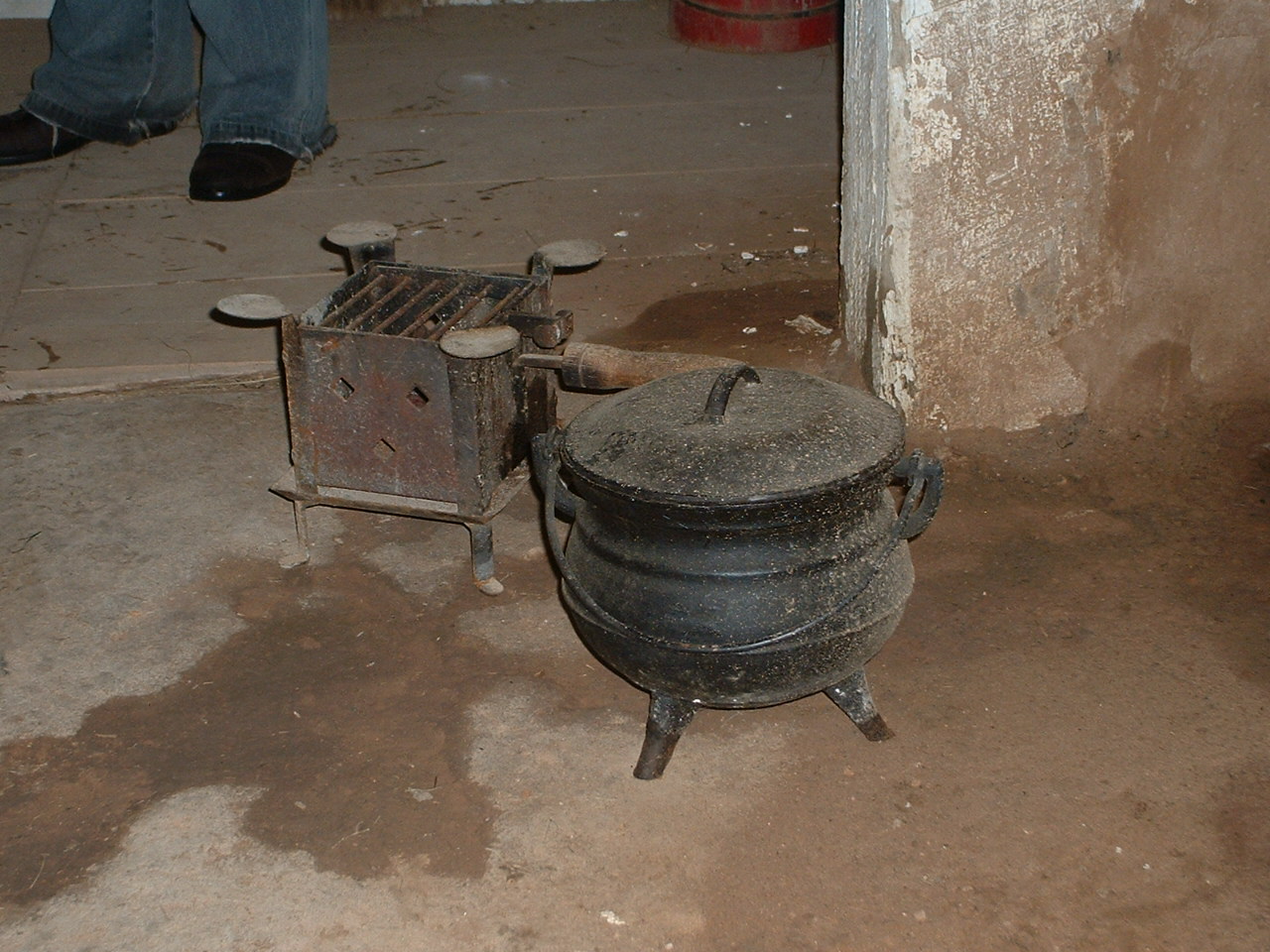This image captures the interior of an old, worn building characterized by a dirty, brownish-gray, and tan concrete floor. The setting includes visible debris and potential wet spots, particularly near the lower middle section of the photograph. Centered in the image is a black, three-legged, cast-iron pot with a lid and side handles, evoking a vintage feel. Adjacent to it, slightly to the left and behind, stands a rusted, square metal object on four legs, featuring a top grill and small discs at each of its corners, with a distinctive grate and a wooden handle protruding from one side. The upper left corner reveals the lower legs of a person, clad in blue jeans with bell-bottom-like cuffs pooling at the ankles, and wearing black shoes, facing towards the left. The background on the right side features a worn, off-white wall, and hints of a red object. Light streams into the room, enhancing visibility despite the overall sense of neglect and age.